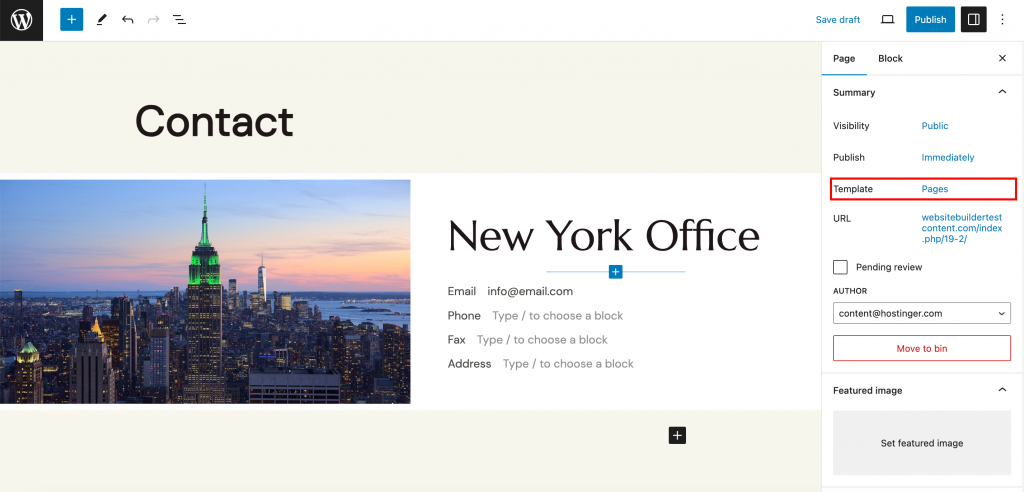**Detailed Caption:**

The image depicts a typical WordPress content management system interface, specifically focusing on the editing screen of a blog post or page. In the top left corner, various administrative options are visible, including "Save Drafts" and "Publish." Tabs for Page, Blog, Summary, and Visibility are displayed, offering different functionalities for content management. The section shows settings for "Publish Immediately" alongside a template selector. 

Additionally, there's a visible URL structure (http://Content.com/index.php/19-2/pending-review) indicating a content review status.

Administrative tools for Wordpress are shown, including a "Featured Image" section where users can set a thumbnail for the post. Centralized contact information lists New York office details, including an email address (info@email.com) and phone numbers, with placeholders prompting users to "type forward slash to choose a blog" for fields like fax and address. 

The interface reflects standard content management operations, integrating plugins or extensions like "HostingGuard.com" and fields related to content authorship.